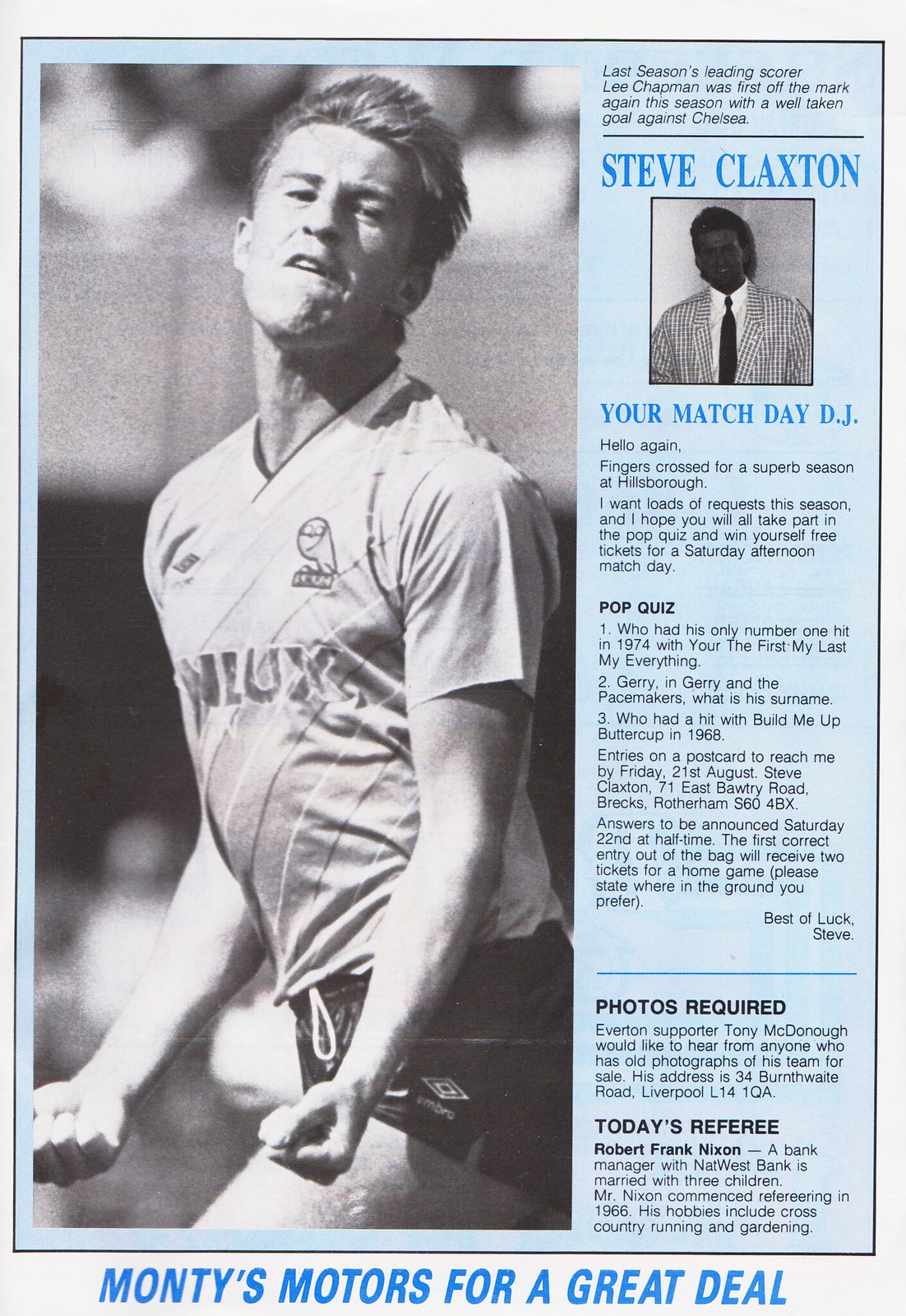The image depicts a page from a magazine or program booklet, showcasing a combination of sports and local content. The left side features a large black-and-white photo of a young, blonde soccer player in black shorts and a jersey with diagonal stripes, captured mid-motion as he pumps his fists upwards, his expression intense as he bites his lower lip. To the right of this image is text mentioning "last season's leading scorer Lee Chapman" and his goal against Chelsea.

Adjacent to this is another photo of the same individual, now identified as Steve Claxton, dressed in a checkered suit, white shirt, and black tie, labeled as "your match day DJ." Below his picture, a message from Claxton invites fans to participate in a pop quiz, requesting song favorites and featuring questions such as "who had his only number one hit in 1974 with 'You're the First, My Last, My Everything'?" and other trivia. There are also details on how to submit quiz entries and win tickets for a Saturday afternoon match.

Further down, in bold, black font, is a section titled "Photos Required," seeking vintage photos of the Everton team, with contact information for Tony McDonough. Additionally, there's a section on "Today's Referee," highlighting Robert Frank Nixon, a bank manager and dedicated referee since 1966, mentioning his hobbies of cross-country running and gardening.

At the bottom of the page, a small advertisement in blue font on a gray background promotes "Monty's Motors for a great deal." The layout and content suggest it might be part of a game day program, combining sports updates, entertainment, and community notices.